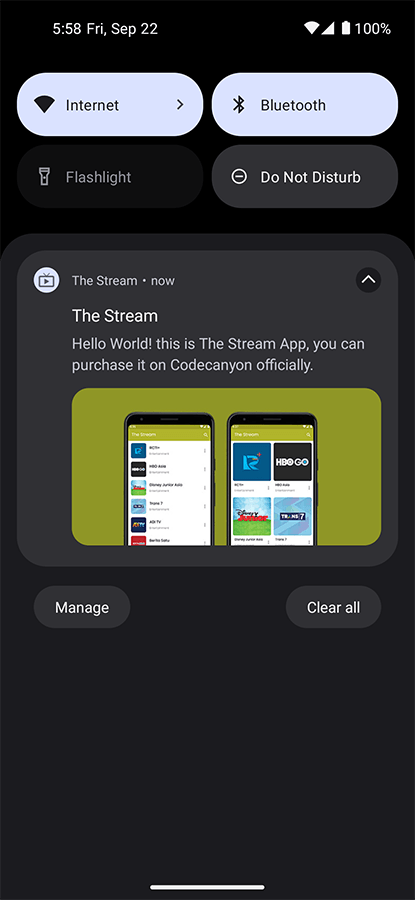**Detailed Caption:**

The screenshot captures the interface of a smartphone with a completely black background. In the upper left corner, white text displays the time "5:58" and the date "Friday, September 22nd." On the upper right side, various status icons are present, including the Wi-Fi signal, cell signal, battery icon, and the battery percentage, which is at "100%."

Directly below the status bar, two buttons are visible. The left button is labeled "Internet," and the right button is labeled "Bluetooth." These buttons have a light background with black text, indicating they are activated. Below these, two more buttons are displayed: "Flashlight" on the left and "Do Not Disturb" on the right, both with a black background and white text, suggesting they are inactive.

Further down, a large tile reads "The Stream" and "Hello World. This is the Stream app you can purchase it on CodeCanyon officially." Within this tile, there is an image showcasing the app and the CodeCanyon website, featuring two smartphones displayed back-to-back with different screens.

At the bottom of the screenshot, two additional buttons are located: "Manage" on the left and "Clear All" on the right. The elements and layout provide a comprehensive overview of a section of the smartphone, with clear indications of active and inactive states of various features.